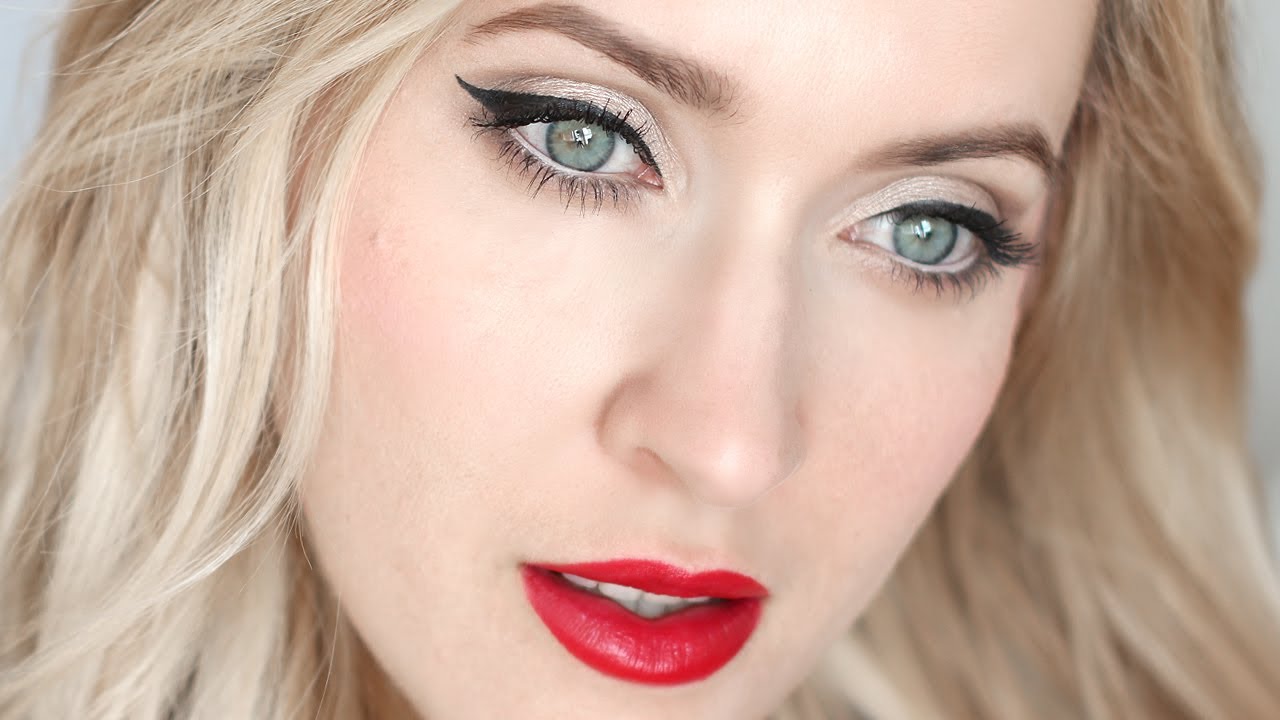The image depicts a close-up of a young, very beautiful Caucasian woman, approximately 28 years old, with striking features. Her long blonde hair appears slightly windswept and frames her face, which fills the majority of the screen, though the image is cropped from about her eyebrow level to just past her lower lip. She is wearing vibrant red lipstick that draws attention to her partially open mouth. Her eyelashes are long and enhanced with heavy mascara, complementing the eyeshadow and eyeliner that accentuate her light-colored eyes, which are described variably as hazel, icy gray, or light green. Her thin eyebrows are shaped and curve upwards. The woman's intense, concentrated gaze is directed downward, possibly at a cell phone or similar object, suggesting she is deeply focused on what she is reading or observing. The background is plain white, adding to the focus on her meticulously made-up face, potentially for a makeup advertisement.